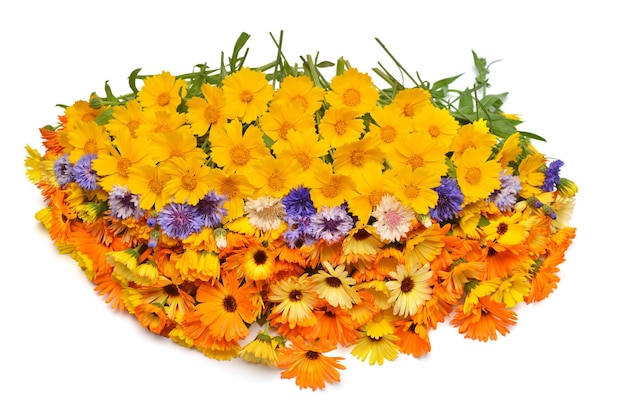This photograph features a meticulously arranged bouquet of flowers against a pristine white background. From a top-down perspective, the arrangement consists of three distinct rows. The bottom row showcases larger daisies in vibrant shades of orange and yellow, each with a deep brown center. Directly above, there's a narrow band of flowers displaying a delicate array of purples, lilacs, and whites—each sporting numerous small petals intermingled to form a striking mid-section. The top layer is composed of medium-sized yellow daisies, their cheerful petals uniformly facing up. Visible green stems extend from the top row, seemingly anchoring the entire composition and adding a subtle touch of natural elegance. This layered, tightly-packed floral display ensures no gaps between the blooms, creating a lush, continuous tapestry of color and texture.